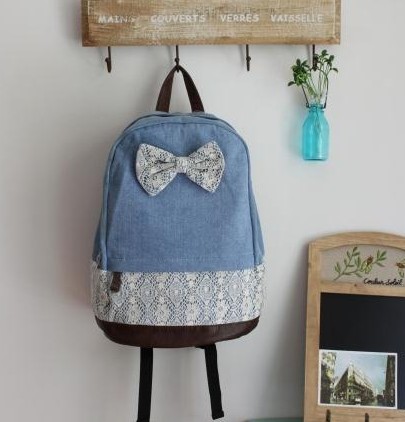In this home entryway scene, a wooden, weathered, four-hook hanger is mounted on a white wall. The wood has a distressed appearance and features four words painted in white, presumed to be in French. From the second hook on the left, a blue backpack hangs by its loop. This backpack is adorned with a white and black bow tie on its exterior, and below the blue top, it has a white and black patterned section, as well as a black bottom with two black straps. The first and third hooks are empty. The fourth hook on the right holds a light blue glass bottle with green plants growing out of it. In the bottom right of the image, there is a small chalkboard with a wooden frame, depicting an art piece of plants at the top and a picture of buildings below.